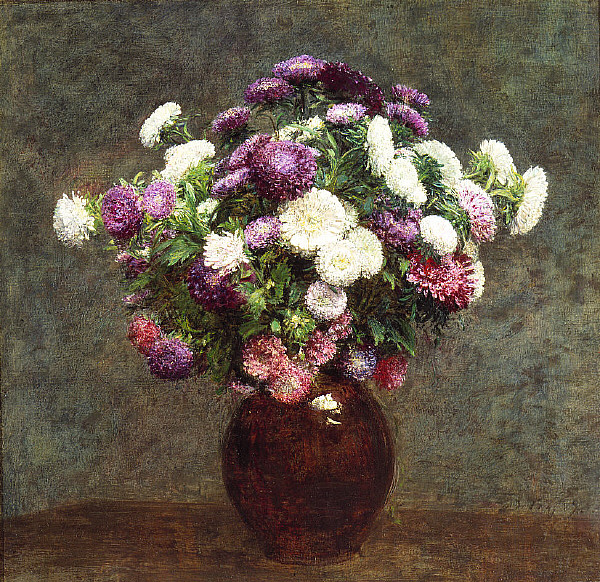This detailed and extremely realistic painting depicts a rounded, shiny vase, predominantly dark brown or reddish-brown in color, placed on a plain brown table surface. The setting is framed by a textured gray background, adding a sense of depth and age with its varied shades and subtle, cracked appearance. The vase, possibly ceramic, appears almost overflowing with a profusion of around fifty flowers, which are primarily white, reddish-pink, and purple. Notably, white flowers dominate the center, while reddish-pink flowers are more conspicuous at the top and sides, and the purple flowers are prominently positioned at the top. Interspersed among the flowers are abundant green leaves, adding to the lush and vibrant composition. Despite lacking an artist's signature, the painting's intricate brushstrokes and nuanced tones contribute to its rich texture and strikingly lifelike presentation.